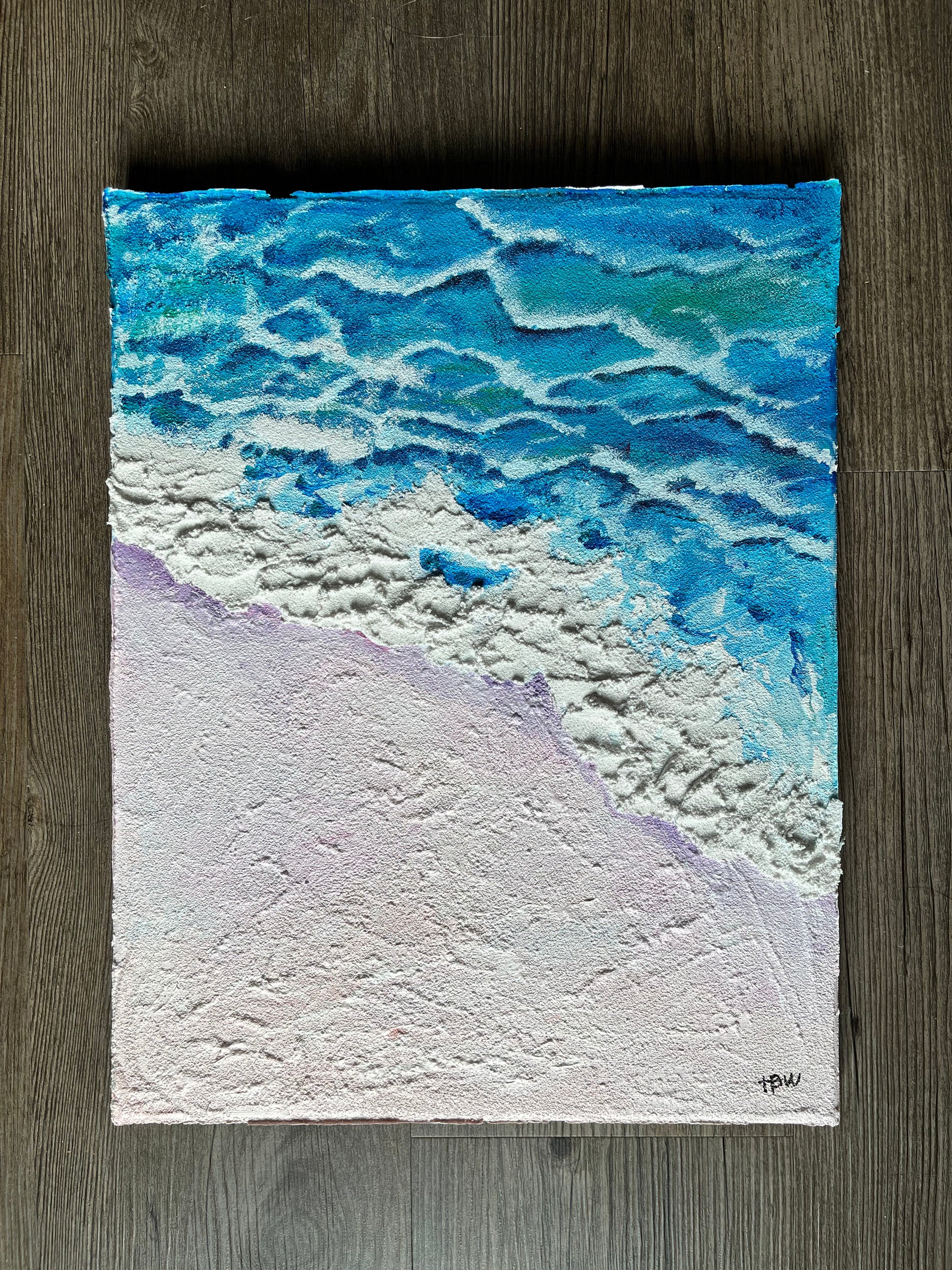This image showcases a textured painting on a dark brownish-gray wooden surface, likely a table or floor, composed of paneled wood. The large rectangular canvas in the center depicts a beach scene with a vivid and realistic portrayal. In the bottom left corner, there's a textured area that mimics tan sand, using raised materials to enhance its realistic feel. Extending from the top right corner, blue and green ocean waves crash onto the sandy shore, with their white foamy edges full of depth and detail. The painting's intricate texture provides a three-dimensional quality to both the water and the sand. Adding a hint of color diversity, there's a small touch of purple embedded in the sand. The painting is signed in black by the artist, with initials that appear to be TBW, located in the bottom right corner of the artwork.